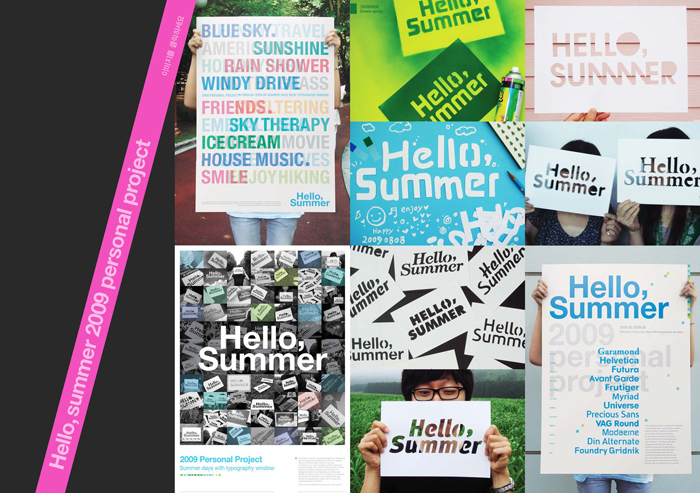This photograph captures a vivid collage of posters, prominently showcasing the phrase "Hello Summer" in various styles and colors. The composite image is set against a black backdrop with a lilac banner running vertically along the left side, reading "Hello Summer 2009 Personal Project" in white text. Central to the collage is a large poster held by a person, featuring a diverse collection of cheerful phrases like "Blue Shine," "Travel America," "Sunshine," "Hope," "Rain Shower," "Windy Drive," and more, concluding with "Hello Summer" in the bottom right corner. The upper left quadrant of the composite highlights a woman holding a multicolored "Hello Summer" sign with vibrant red, blue, yellow, and green letters. Neighboring this, various "Hello Summer" posters are seen in alternating green, white, pink, and blue hues. The lower sections include another series of "Hello Summer" signs in varying fonts and stickers, tagged as "2009 Personal Project." To the middle right, a person holds a monochromatic "Hello Summer" sign, surrounded by smaller versions of the same phrase. Finally, the bottom right features a person holding another detailed poster adorned with typographies labeled Garamond, Helvetica, Futura, among others, forming a structured yet eclectic representation of summer's welcoming theme.